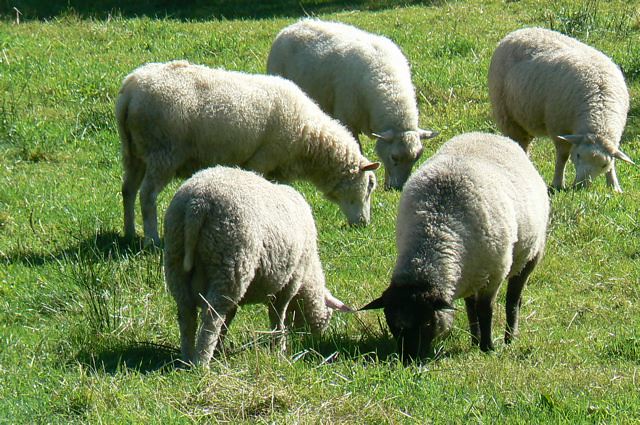In this sunlit photograph, a picturesque scene unfolds with five pudgy sheep grazing in a field of naturally growing light green grass, interspersed with some yellowing patches. The sheep, all adorned in full wool coats, have their ears pointed outward as they intently munch on the grass with their heads bent down. Four of the sheep are predominantly white, while one distinctive sheep in the front-right of the image stands out with its black face, black ears, and black legs. The sheep form a loose semi-circle, except for the black-faced one which is turned slightly towards the viewer. A smaller sheep can be seen on the left side of the image. The background reveals a gentle, expansive grassy valley, partially obscured by a shadow—possibly cast by a tree or a building—at the top left corner of the image. The scene captures a tranquil, pastoral moment amidst the quiet splendor of a warm day in the countryside.